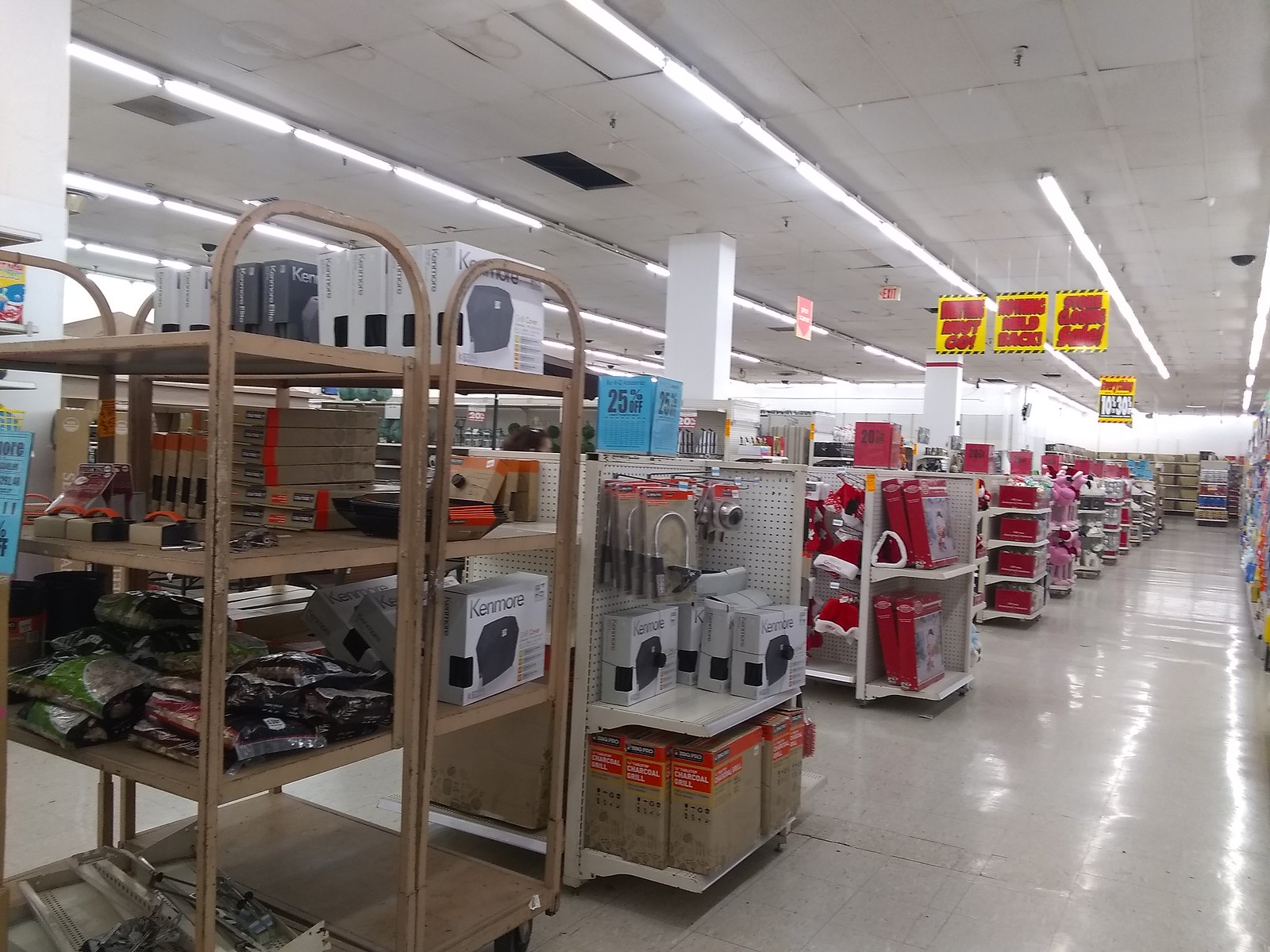The photograph captures the interior of a moderately large big-box store, showcasing a diverse array of merchandise typical of a discount, multipurpose retailer. The store features modular shelving units organized in long aisles, with end-of-aisle displays and banners hanging from an acoustical tile ceiling equipped with fluorescent lights. The well-lit space, marked by parallel lines of bright illumination, has a well-worn tile floor, indicating high foot traffic. Prominently, there is a Kenmore box, suggesting the sale of electrical appliances, placed on a trolley perhaps used for restocking. Nearby, bags of various items are mixed alongside Kenmore products, and further down the aisle, a clip-on lamp with a gooseneck arm is advertised at 25% off. At the store's left side, wooden or wicker shelving, stacked four levels high, hold a mixture of items in both bags and boxes. Light support pillars are visible throughout the space, reinforcing the industrial, functional ambiance. The store exudes a budget-friendly atmosphere, evident from the eclectic range of goods and the utilitarian store fittings.